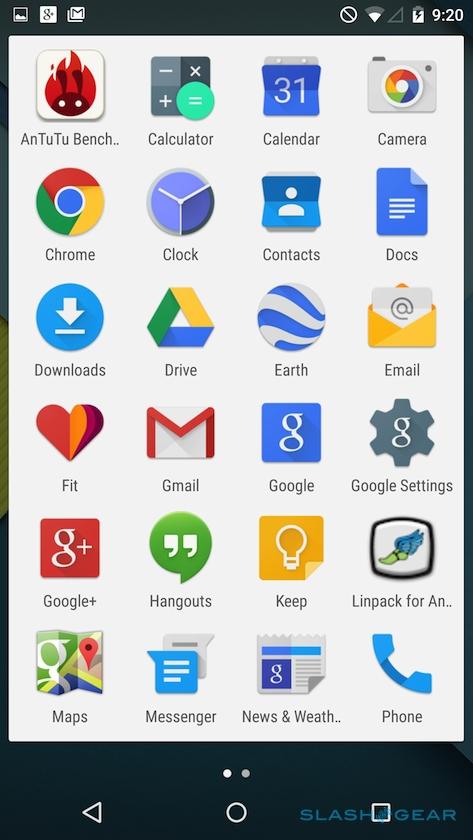Displayed on the cell phone screen is a detailed interface. The top section of the screen features a black status bar containing various icons: a Gmail notification in a white square on the left, and several system indicators on the right, including a "Do Not Disturb" circle with a diagonal line, Wi-Fi signal bars (no cell signal bars visible), and a battery icon showing the device is charging with the time displayed as 9:20.

Below the status bar, the majority of the screen showcases a white background filled with six rows of four app icons each, totaling 24 icons. These icons, appearing orderly in a 4x6 grid, include:
- AnTuTu Benchmark
- Calculator
- Calendar
- Camera
- Chrome
- Clock
- Contacts
- Downloads
- Drive
- Earth
- Email
- Fit
- Gmail
- Google
- Settings
- Google+
- Hangouts
- Keep
- Linpack for Android
- Maps
- Messenger
- News & Weather
- Phone

At the bottom of the screen, just above the navigation bar, there are two dots and a circle, indicating the presence of another page of icons.

The navigation bar itself, positioned at the very bottom, includes a back arrow on the left, a circular home button in the middle, and a square button on the right, which may denote recent apps.

Overlapping the app grid, in a green-colored overlay, the text "SlashGear" is displayed prominently. The background beneath this overlay is a mix of purple, blue, red, yellow, green, gray, black, and white hues.